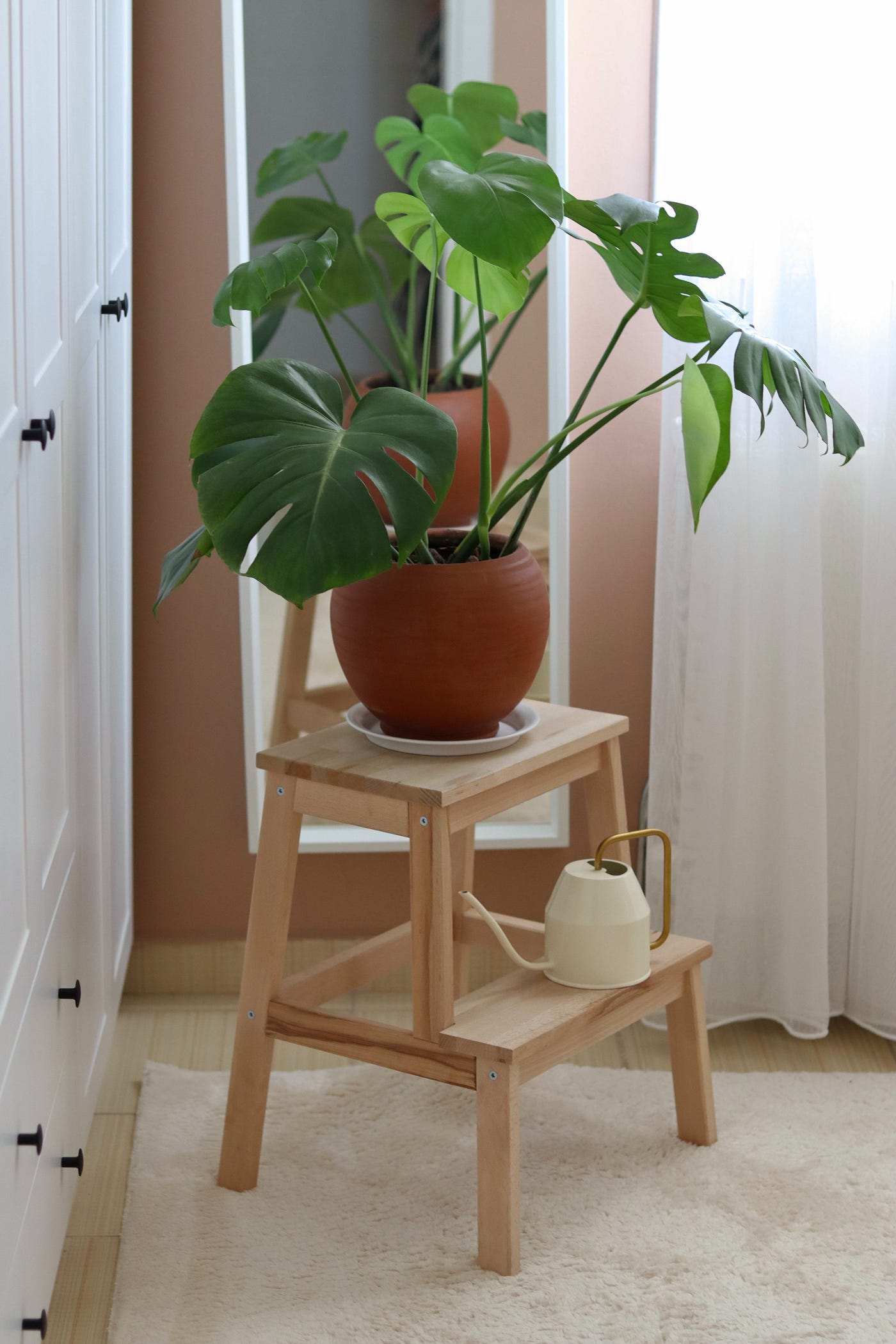The image depicts a close-up angled view of a wooden plant stand that resembles a step stool placed in a residential room. The stand, crafted from light-colored wood, features a longer bottom shelf and a shorter top shelf. On the bottom shelf sits a small white metal watering can with a bronze handle. The top shelf holds a single round terracotta planter with large, green elephant ear plants, set on a small white plate. This arrangement is resting on a cream-colored carpet in front of a tan-colored wall. A sheer white floor-length curtain is visible to the right, while to the left, there's a white wooden closet door with black fixtures. A white long mirror in the background reflects the plant, giving the illusion of more greenery. The overall scene is suggestive of a cozy and well-decorated living space.